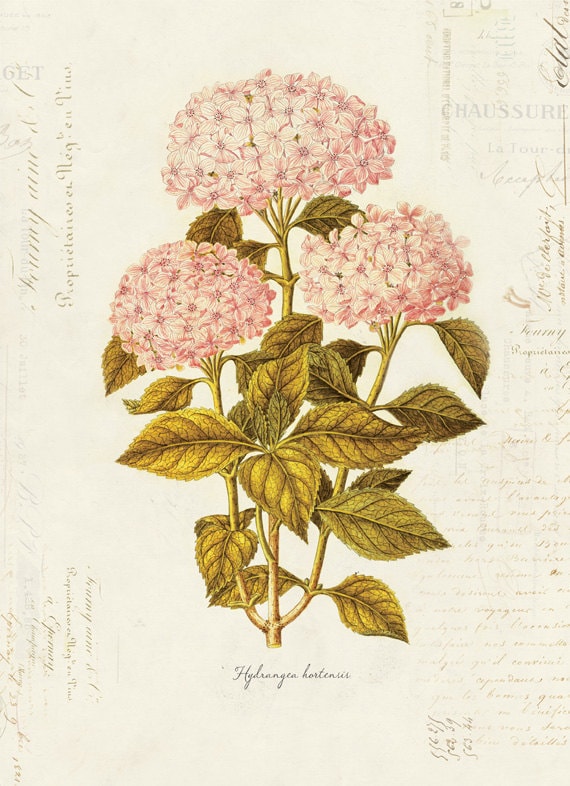This detailed image showcases a botanical illustration of three pink hydrangea blooms, each perched atop separate stems adorned with light green to greenish-gold leaves that resemble mint leaves—oval, slightly rugged, and pointed at the ends. The backdrop is a stark white, overlaid with a flurry of cursive scripts and handwritten notes that meander through the margins, creating a textured and vintage feel reminiscent of an old-time flower book or postcard. At the base of the illustration, the Latin name "Hydrangea hortensis" is inscribed in small, elegant script, adding a scholarly touch to this aesthetically pleasing and informative image.